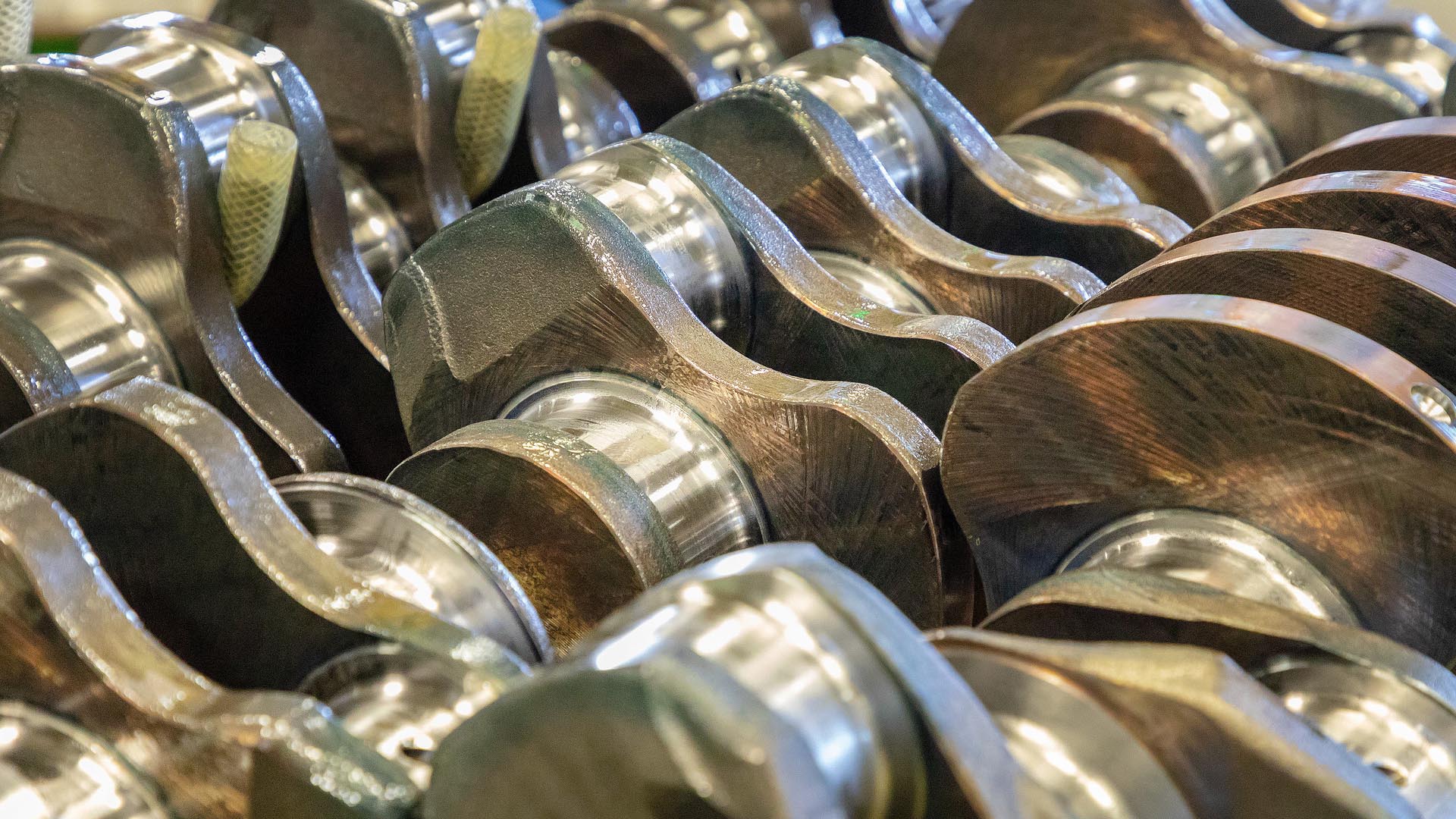This image is a detailed, zoomed-in photograph of intricate, industrial machined metal parts, potentially from a motor or engine. Prominently featured are several round, kidney-shaped, thick metal plates with embedded round drums. These appear rusty and somewhat aged. Between these plates are camshaft-like structures, aligned side by side. In the upper left corner, two ribbed plastic tubes, with a distinct cross-hatched pattern, extend outward and loop down, indicating a complex layout of hoses that are not connected to any specific part, hanging freely in the background. The metal components show signs of etching, not for decoration, but as a result of the machining process, and the lighting highlights the smoother surfaces while the etched areas remain subdued. This setup suggests it is part of a larger, stationary industrial machine.